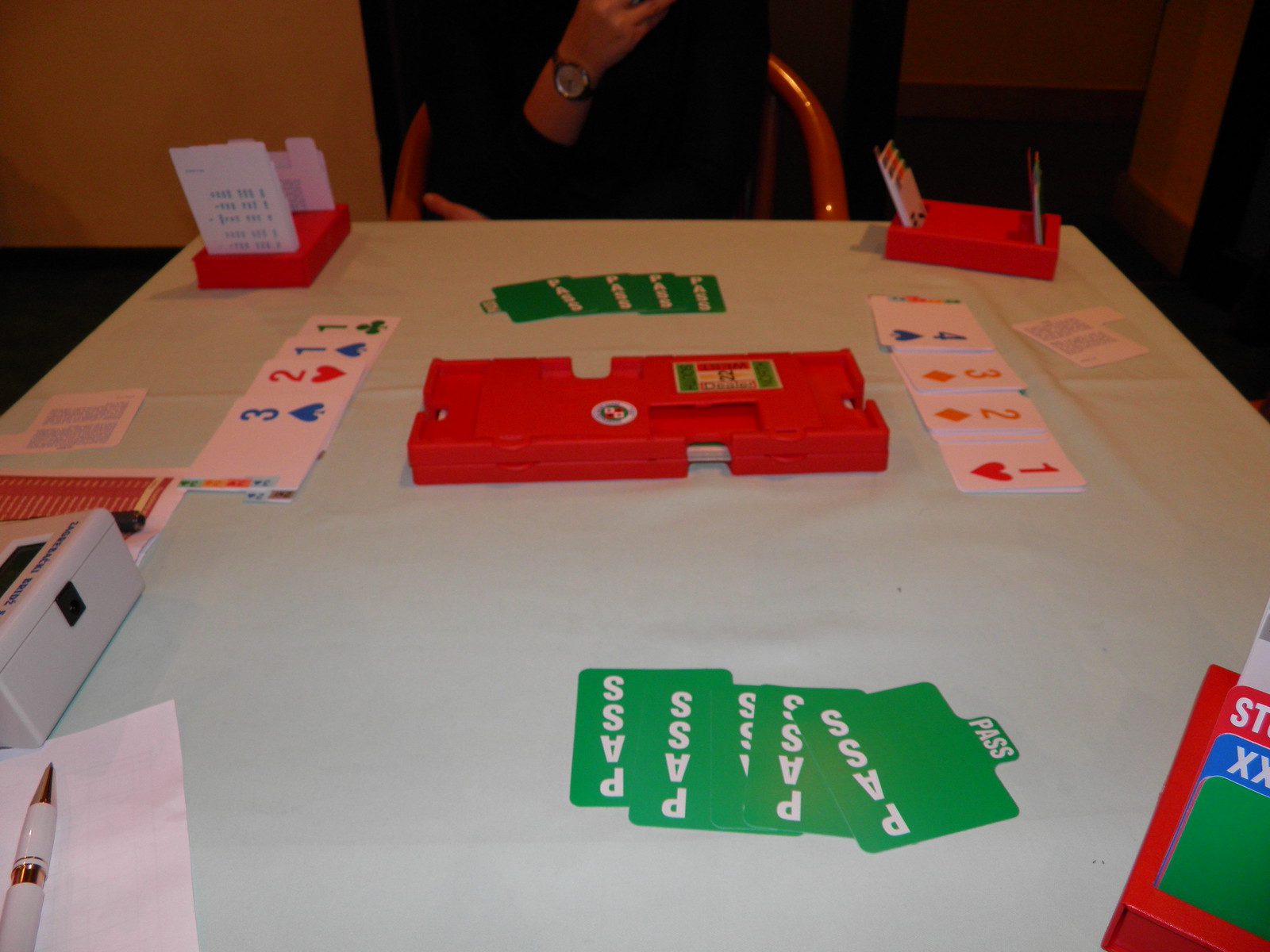In this lively image, several individuals are engrossed in a card game spread across a large table. Dominating the center of the table is a prominent red plastic contraption, possibly a card shuffler or dispenser, which seems to be an essential element of the game. Alongside this contraption, various cards are scattered with distinctive colorful designs: blue spades, yellow diamonds, red hearts, and green clubs. Notable card denominations like the Four of Spades, Three of Diamonds, Two of Diamonds, and Ace of Hearts are visibly spread out.

Towards the top of the picture, a person's hand, adorned with a wristwatch, is raised to their face, although their face remains out of view. The mystery card player's hand hints at a moment of contemplation or decision-making within the game.

Directly in front of the camera and across the table, five green cards with the word "PASS" emblazoned in white letters are neatly arranged, mirroring a similar setup for another player who appears to have four such cards. Additional red plastic contraptions, filled with cards, are seen at the table’s top left and right corners, further emphasizing the game's complexity.

In the bottom left corner, a pen rests on a piece of paper, suggesting that scores or game notes are being diligently recorded. The vibrant colors of the cards and the eclectic array of gaming paraphernalia create an intriguing and engaging scene, capturing the focused energy of the players.